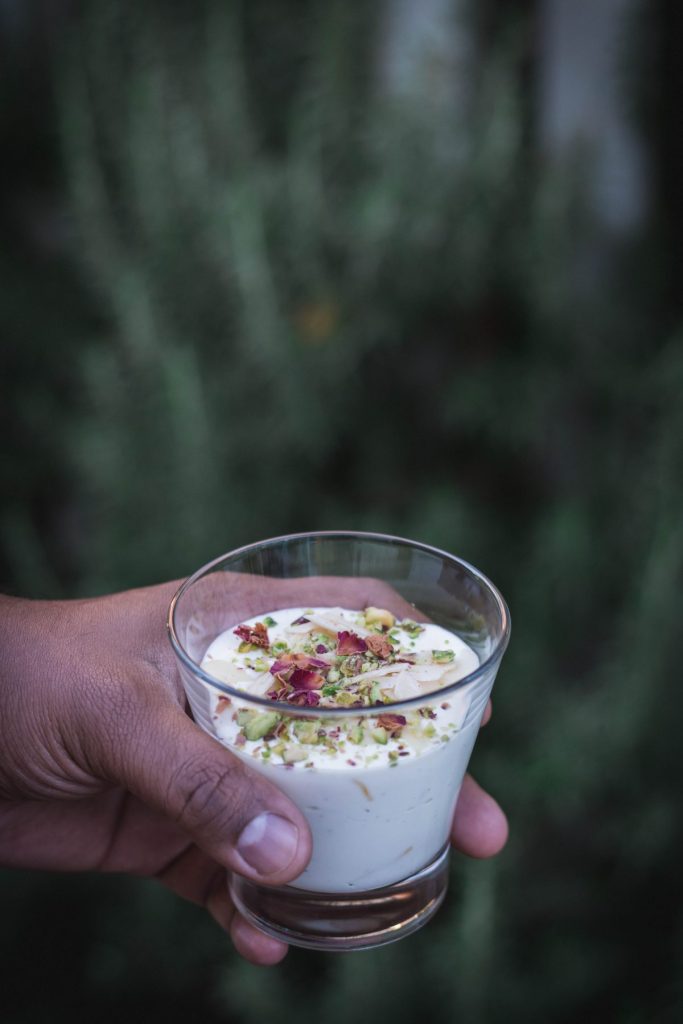A brown-skinned hand emerges from the left side of the image, holding a short glass cup in the lower center of the frame. The hand, identified as the left hand due to the visible thumb and pinky below the cup, features short nails. The cup contains a white liquid or substance, possibly yogurt, custard, or a dip, adorned with colorful toppings in shades of maroonish red, light green, yellow, white, and purple. The glass is round at the bottom with a wider opening at the top, reflecting light on both the hand and its lower part. The blurred background showcases dark green vegetation, adding a natural element, though it's unclear whether the setting is indoors or outdoors, or if it was taken during the day or night. The focal point of the image is clearly the glass and its vibrant contents.